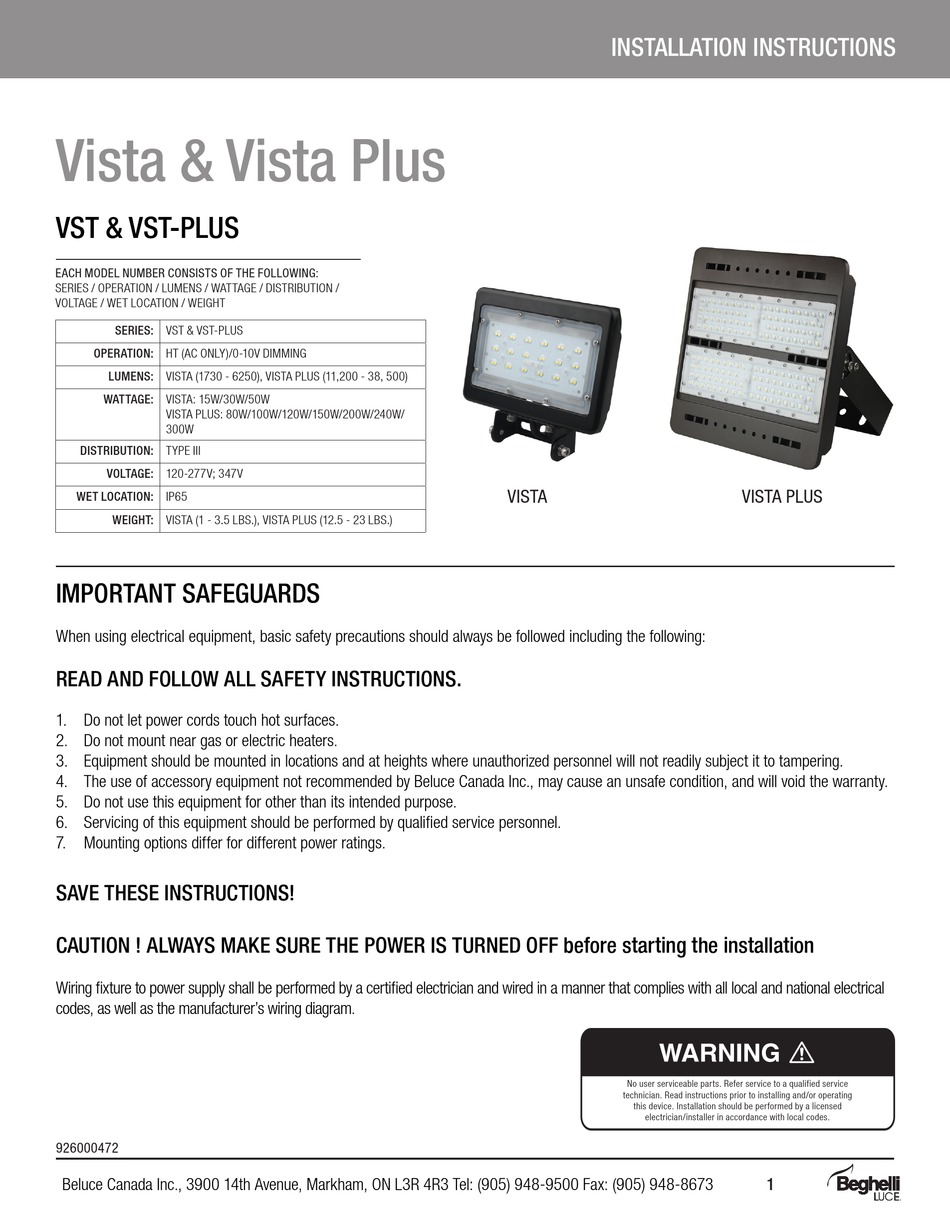This image is a screenshot of a product advertisement for "Vista" and "Vista Plus," prominently displaying installation instructions. The top section of the flyer has a gray background, with white text on the top right corner reading "Installation Instructions." The top left corner features the product names: "Vista" for the smaller device and "Vista Plus" for the larger device.

The advertisement includes images of both products, each mounted on stands. The smaller device, named "Vista," is shown on the left, while the larger device, named "Vista Plus," is positioned on the right.

The middle section of the flyer provides critical safety and installation guidelines as follows:
1. Do not let power cords touch hot surfaces.
2. Do not mount the equipment near gas or electric heaters.
3. Equipment should be mounted in locations and at heights where authorized personnel will not readily subject it to tampering.
4. The use of accessory equipment not recommended by Blue's Canada Inc. may cause unsafe conditions and will void the warranty.
5. Do not use this equipment for purposes other than its intended use.
6. Servicing the equipment should be performed by qualified service professionals or personnel.
7. Mounting options differ for different power ratings. 

The flyer emphasizes the importance of reading and following all safety instructions to ensure proper and safe installation of the Vista and Vista Plus products.